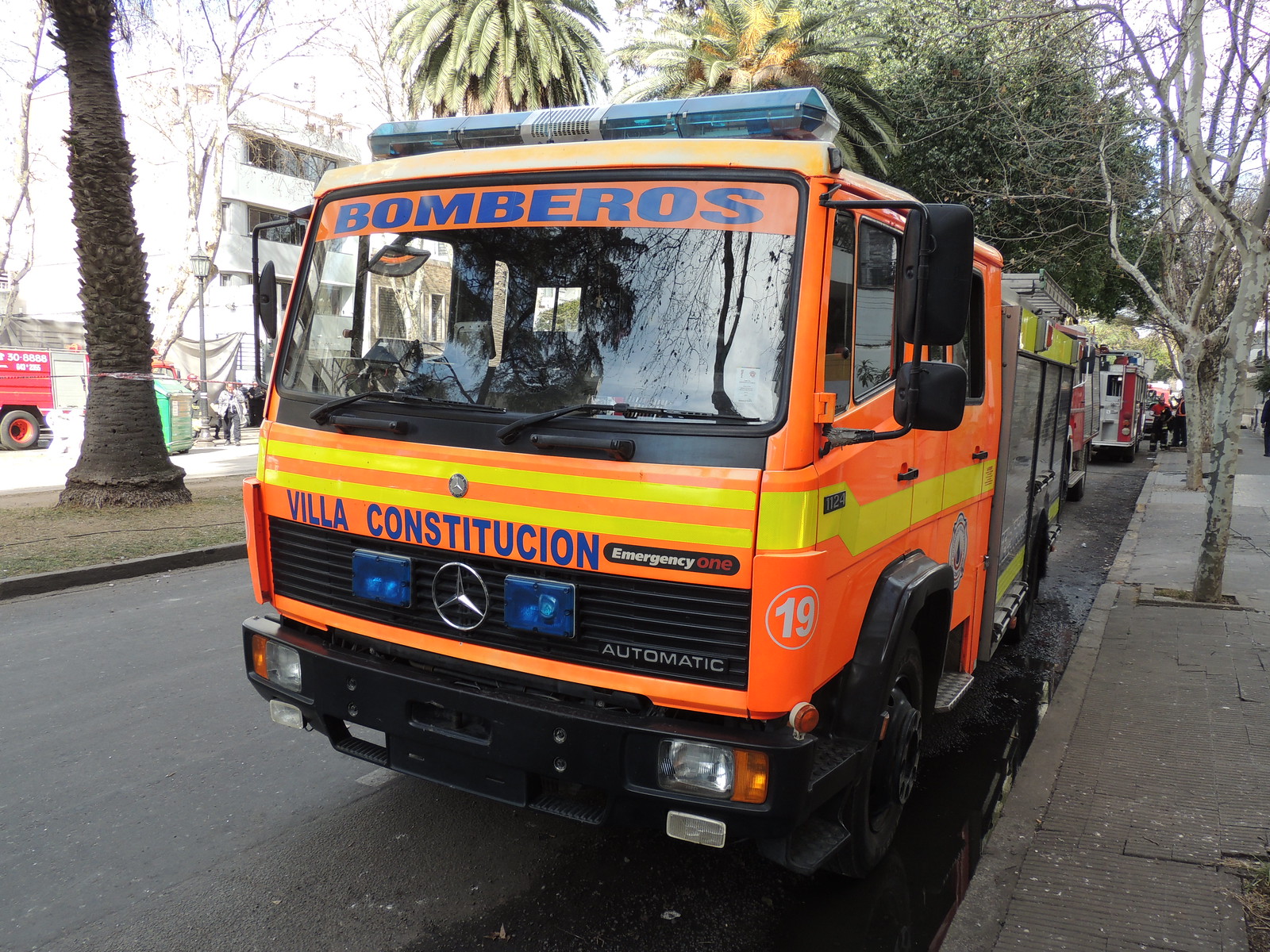Captured in a photographic style, this detailed image portrays an outdoor city street during the day. Dominating the center is an orange and yellow emergency truck, marked "Bomberos Villa Constitución Emergency 1 Automatic" with bands of yellow on the cab and the distinctive Mercedes-Benz logo on the front. Blue emergency lights adorn the top of the cab, and the number 19 is visible in the right-hand corner. Parked on the black asphalt street, the truck is accompanied by other commercial vehicles, including what appears to be a red fire engine in the background.

To the left of the truck, a tree with a leaning trunk stands amidst other green-leaved trees, while to the right, the sidewalk hosts more leafless trees and several pedestrians. Across the street, a line of trees, including some palm trees, frames a multi-story gray concrete building. A median separates this scene from another road visible on the left side of the image. The environment, populated with various colored objects - gray, black, orange, yellow, blue, silver, and red - signifies a bustling downtown area at midday.